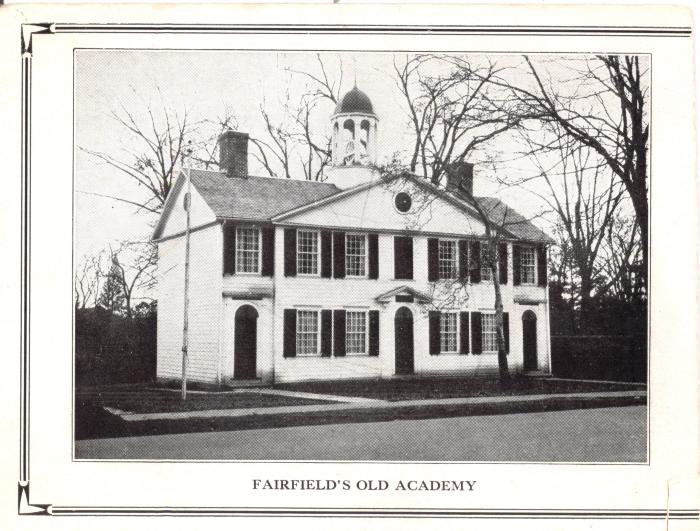The photograph depicts Fairfields Old Academy, captured in a vintage, black-and-white style with a strong sense of antiquity. The image is set within a stylized black line border on a white background, creating a framed effect. At the bottom of the white border, black text reads "FAIRFIELDS OLD ACADEMY."

The image showcases a grand, two-story building viewed from the street. The building's facade is characterized by three doors, each set beneath an archway, flanked by numerous windows with small glass panes framed in white. At the roofline, two chimneys tower on either side of a central dome-like structure. This dome is an eye-catching architectural element supported by arches and columns, crowned with a spire.

The photograph extends to the surroundings, with grass visible in the front yard and several trees framing the scene on both sides. The overall aesthetic of the image accentuates the historical and stately nature of Fairfields Old Academy, suggesting its erstwhile usage as an old schoolhouse. The dominant hues are variations of black, white, and gray, reinforcing the image's vintage feel.